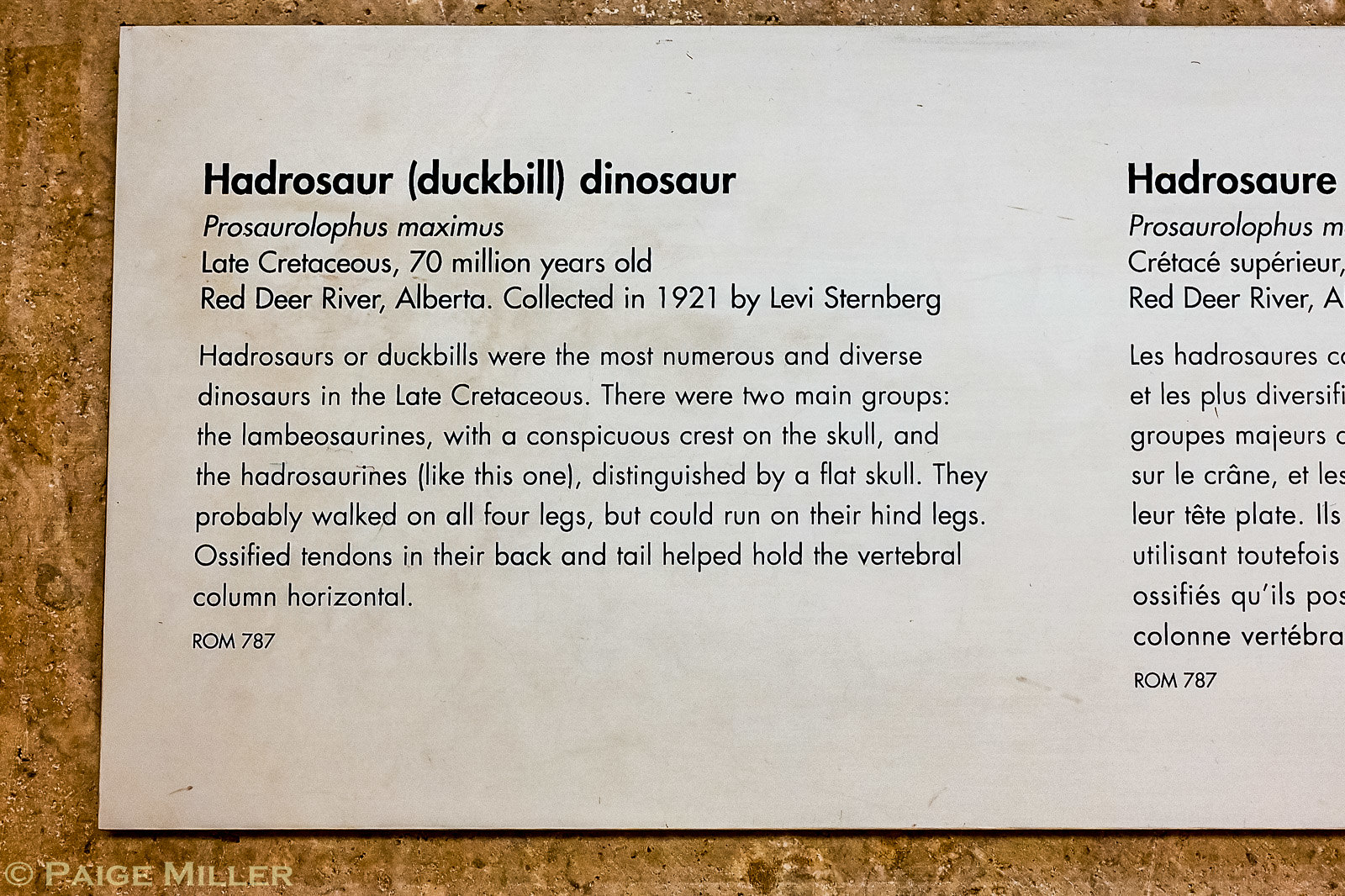The image displays a horizontally oriented piece of paper, approximately 13 by 9 inches in size, featuring bold black text. At the top, it prominently states "Hadrosaur" with "duck-billed dinosaur" in parentheses. Beneath this title, the text reads "Prosauroflophus maximus," followed by details: "Late Cretaceous, 70 million years old, Red Deer River, Alberta, collected in 1921 by Levi Sternberg." 

The main paragraph below this introduction explains that Hadrosauruses, or duck-billed dinosaurs, were the most numerous and diverse dinosaurs during the Late Cretaceous period. It specifies that there are two main groups of these dinosaurs: the Lambiosaurines, which feature a conspicuous crest on their skulls, and the Hadrosaurines, like the one described, known for their flat skulls. These dinosaurs likely walked on all four legs but could run on their hind legs. The text further mentions that ossified tendons in the back and tail assisted in maintaining the horizontal position of the vertebral column. At the bottom, the reference "ROM 787" and a copyright notice attributed to Paige Miller are also present.